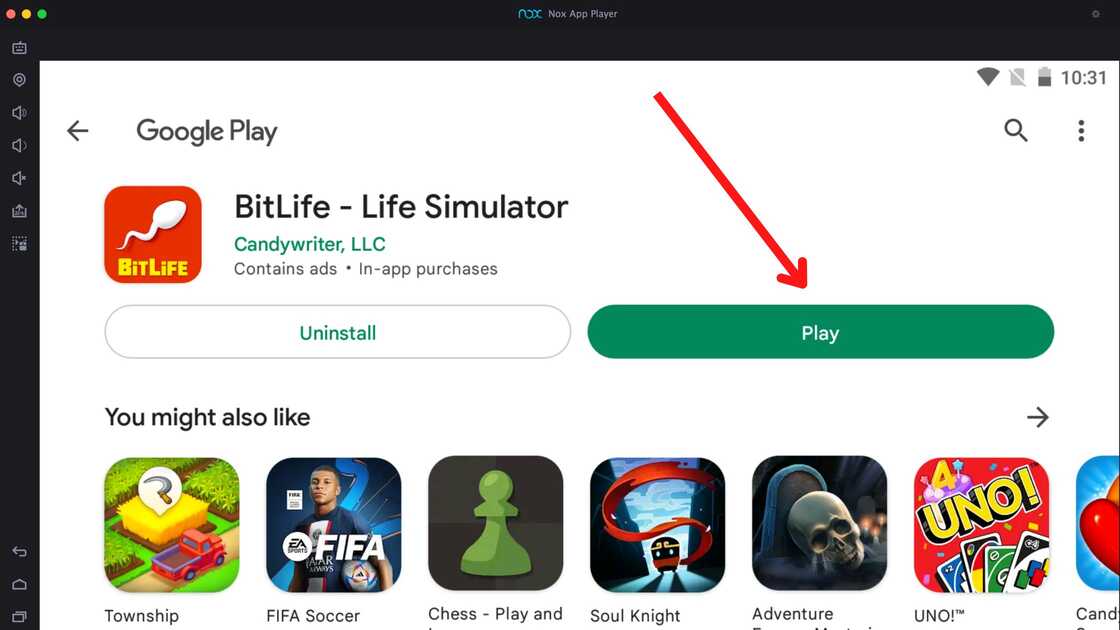The screenshot captures the interface of Knox App Player, an Android emulator, showcasing the Google Play Store. At the top of the screen, "Knox App Player" is clearly displayed. The Google Play Store is open, featuring the app "BitLife - Life Simulator" by CandyWriter, LLC, which includes ads and in-app purchases. The app's icon depicts a sperm cell on a red background with the title "BitLife" below it. 

Beneath the app title and publisher information are two prominent buttons: a white "Uninstall" button with green text on the left and a green "Play" button with white text on the right. A large red arrow points towards the "Play" button, emphasizing its importance.

Further down, there is a "You Might Also Like" section displaying additional app suggestions including "Township," "FIFA Soccer," "Chess," "Soul Knight," and partially visible titles possibly being "UNO" and "Candy Crush." 

On the left sidebar, there are several icons representing different options such as volume control and settings. The top right-hand corner of the Google Play page shows the time as 10:31.